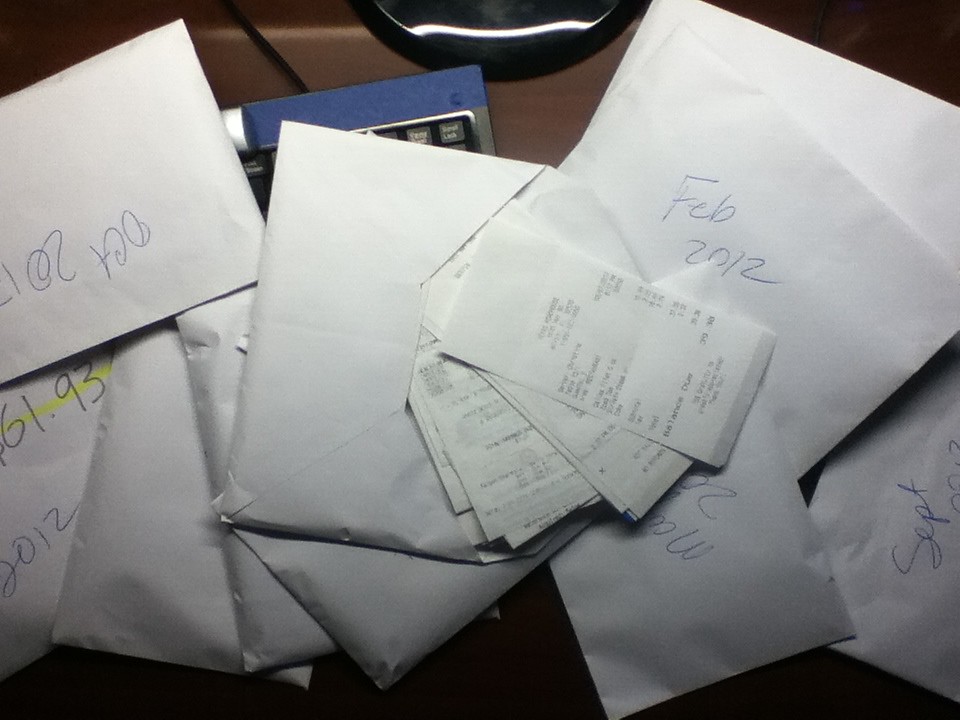This is a detailed photograph of a cluttered desk laden with white envelopes and various receipts, suggesting thorough record-keeping, possibly for tax preparation. A black-and-blue computer keyboard peeks from beneath the scattered envelopes, each loosely labeled in blue ink with different months and years: notably February and October 2012, and some from September. Many envelopes are crinkled and some are flipped open, revealing piles of indistinguishable receipts, with one showing an expenditure of $39. Amidst the chaos, a portion of a calculator or adding machine is visible in the background, along with a shiny, reflective silver object that could be a scale for postage. The photograph conveys a sense of meticulous but haphazard organization, with the person appearing to keep detailed monthly records of purchases for several years.